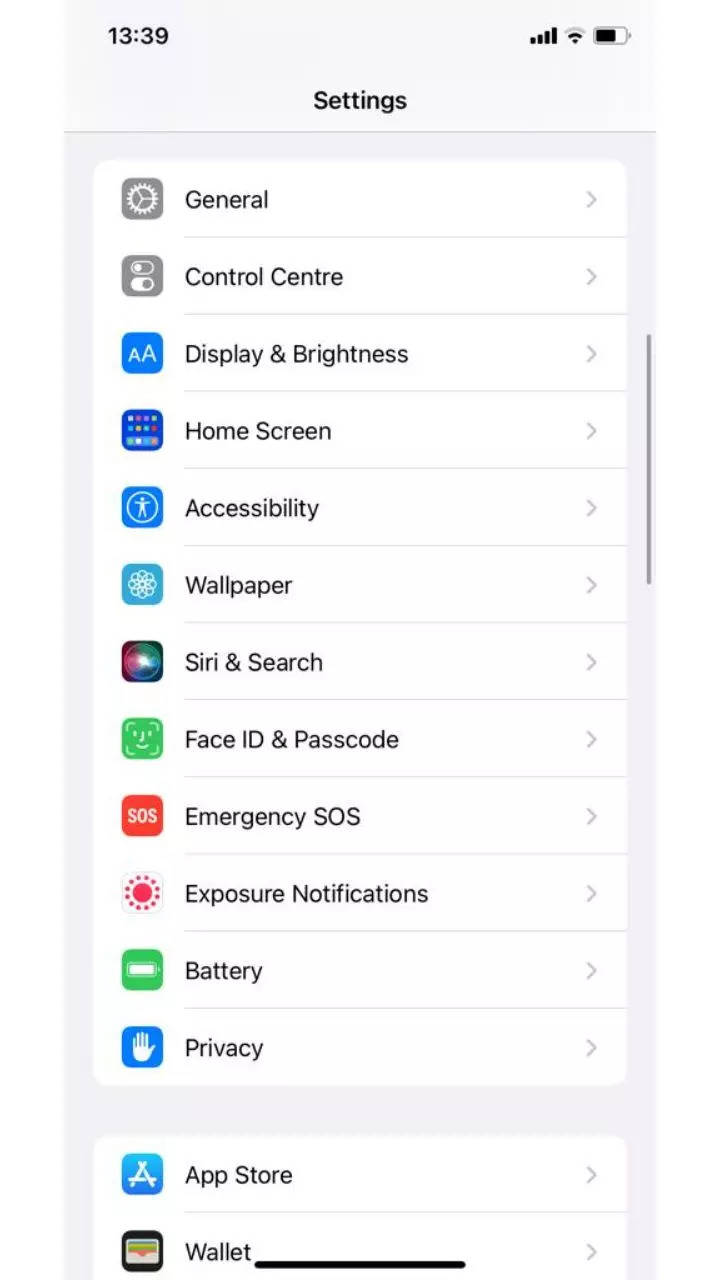The image depicts the settings menu of an iPhone. In the top left corner, the time is displayed as 13:39, and the upper right corner shows the device has full Wi-Fi signal bars and an estimated 80% battery life. The settings menu's header is a black bar labeled "Settings." Below the header, a vertical column of options, each accompanied by icon images on their left, is presented. The options are as follows:

1. **General** - No icon description provided.
2. **Control Center** - No icon description provided.
3. **Display & Brightness** - Icon is a blue square featuring two white "A" letters, one smaller and one larger.
4. **Home Screen** - No icon description provided.
5. **Accessibility** - Icon is a blue square with a white stick figure in a circle, arms outstretched.
6. **Wallpaper** - No icon description provided.
7. **Siri & Search** - No icon description provided.
8. **Face ID & Passcode** - No icon description provided.
9. **Emergency SOS** - Icon is an orange square with "SOS" written in white capital letters.
10. **Exposure Notifications** - No icon description provided.
11. **Battery** - Icon is a green square with a white, fully charged battery symbol.
12. **Privacy** - Icon is a blue square with a white hand symbol, resembling a stop gesture.
13. **App Store** - No icon description provided.
14. **Wallet** - No icon description provided.

The image provides a clear and detailed view of the various settings options available on the iPhone, each visually distinguishable by unique icons.